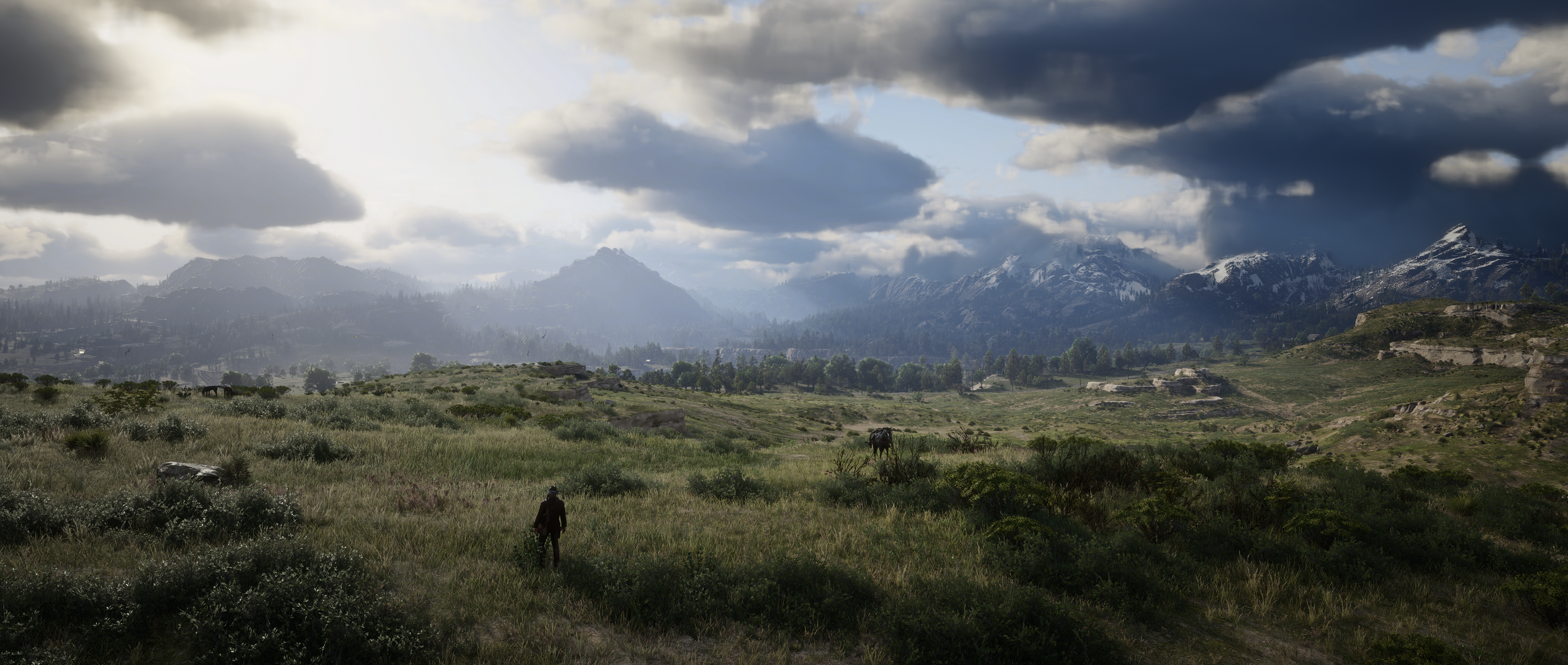A detailed daytime photograph showcases a figure dressed in dark clothing standing solitary in the middle of a sprawling, open field. The green grass in the field varies in height and hue, with patches that are lighter or darker. In the distance, majestic mountains rise, some capped with sparkling snow, lending a serene backdrop to the scene. The sky overhead is heavily clouded, with thick, gray clouds mingling with lighter, almost white ones. Despite the cloud cover, slivers of sunlight manage to pierce through, casting beams of light onto the grass below. Patches of dirt are sporadically visible amidst the lush grass. Tall trees frame the background, adding an extra layer of depth and natural beauty to the landscape.